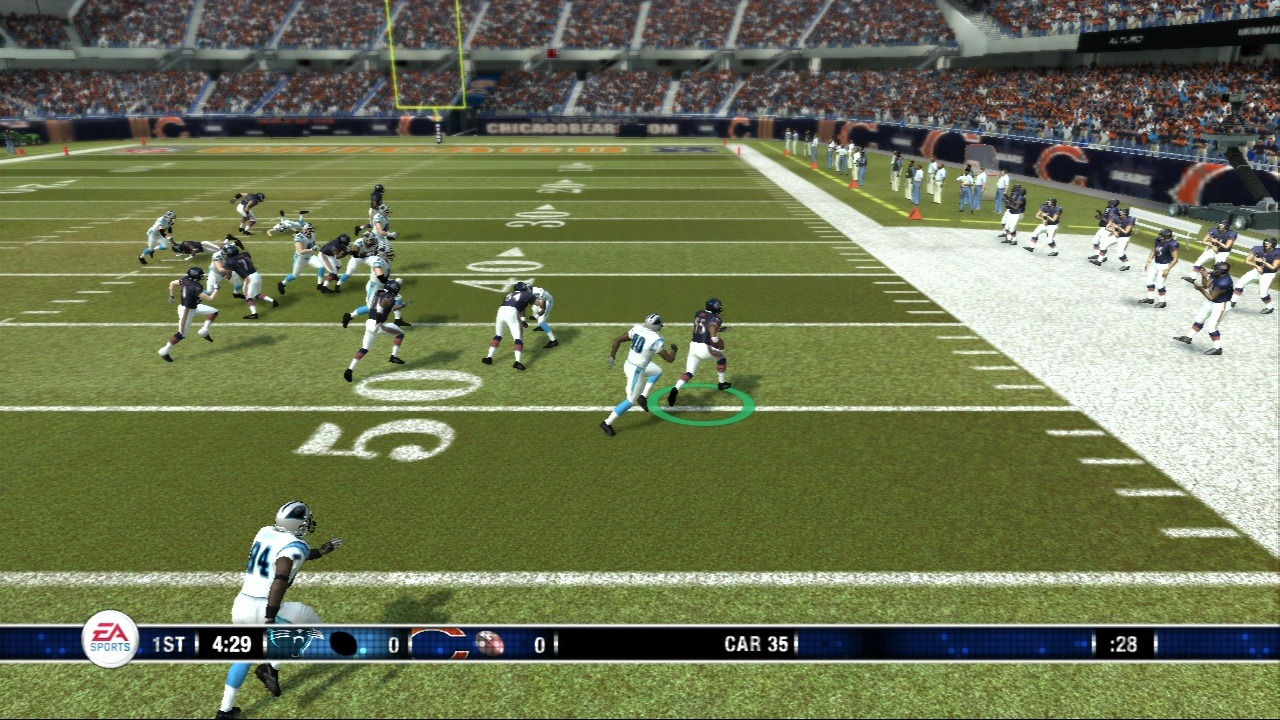In this detailed screenshot from the EA Sports football video game, we are currently in the first quarter with just 28 seconds elapsed, and the score is tied at 0-0. The timestamp on the screen reads 4:29. A player, designated by the number 35 or possibly 351, is highlighted with a green circle, drawing attention amidst the in-game action. The vibrant green astroturf is clearly marked with yardage lines at intervals of 50, 40, and 30 yards. In the midst of a bustling stadium crowd of thousands, another player can be seen running with the ball, setting an anticipatory tone for an imminent play.